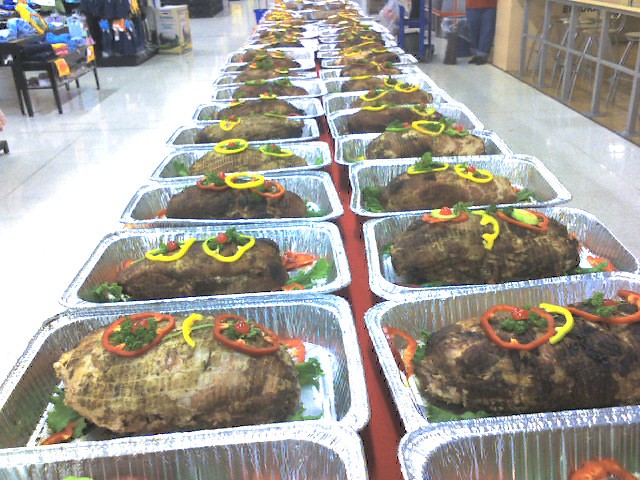This vibrant color photograph captures an extensive buffet set on a long, narrow table draped in a red tablecloth. The table is lined with rows of aluminum foil trays containing generously sized, brown-roasted meats. Each tray is meticulously garnished with cut red and yellow bell pepper rings and sprigs of fresh parsley. There appear to be approximately 15 trays per side, amounting to a striking total of 30 trays that run the length of the table. Chairs are visible at the top right of the image, set against a backdrop of gleaming white tile flooring. The setup suggests a large-scale culinary preparation, possibly for an event like a community feast, charity event, or commercial sale.